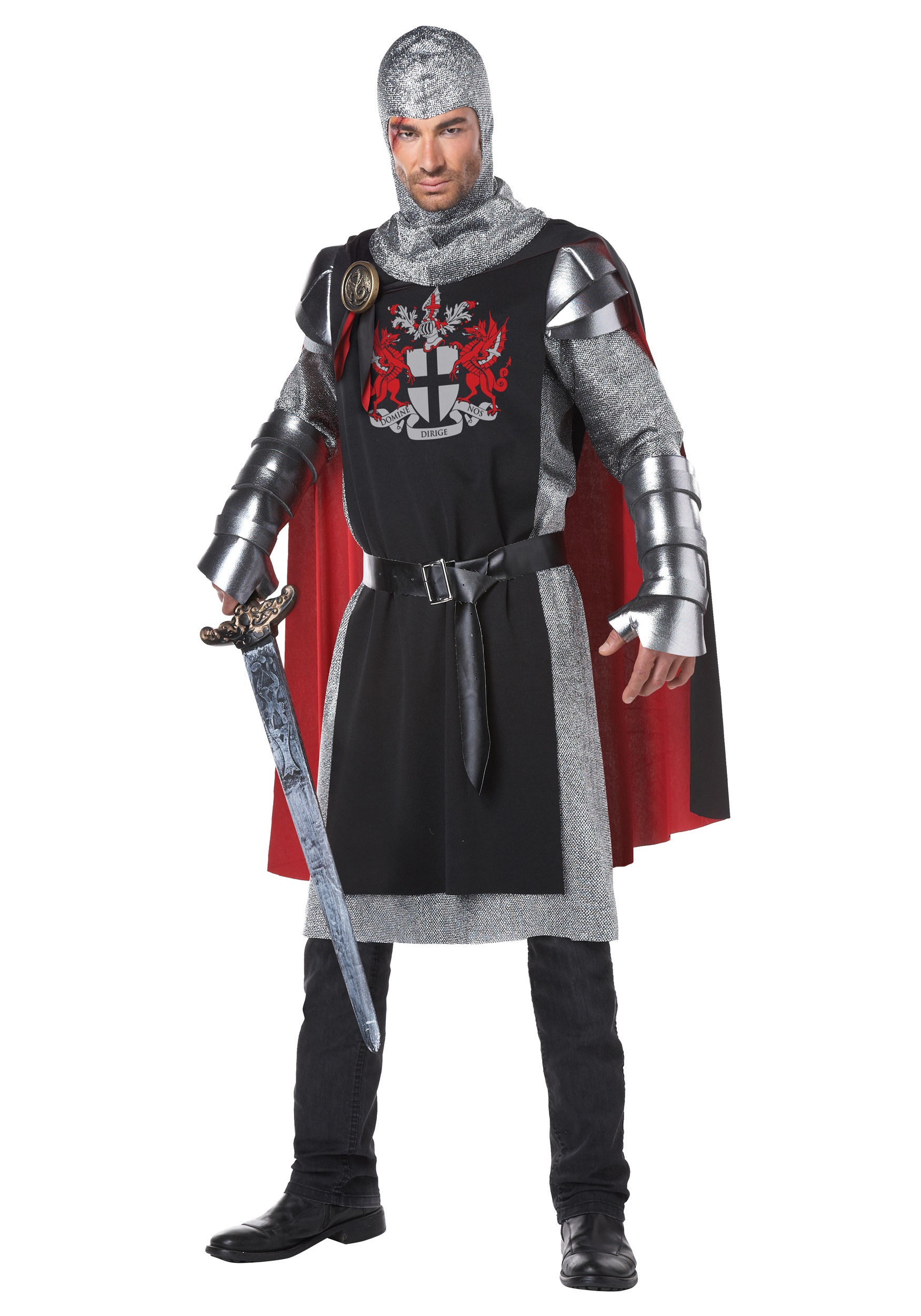The image features a man dressed in a detailed medieval knight costume standing against a solid white background. The man's attire consists of modern black dress shoes and black pants, over which he wears a black tunic or tabard. Under this tunic is a chainmail skirt and chainmail sleeves, complemented by plated arm guards and shoulder guards. His head is covered with a chainmail cowl, adding to the authentic medieval appearance, although it stops short of being a full helmet. The black tunic is adorned with a shield emblem featuring red dragons on either side. He also wears a striking red and black cloak, with a red lining and metallic clasp over one breast. The costume is completed by a belt and a long sword. Additionally, he has a notable scar across his eye, enhancing the warrior aesthetic. The polished silver armor pieces, while seemingly plastic, convincingly mimic real metal armor. The crest on his cloak bears the Latin phrase "Domine Dirige Nos," shaped like a cross and flanked by red beasts.